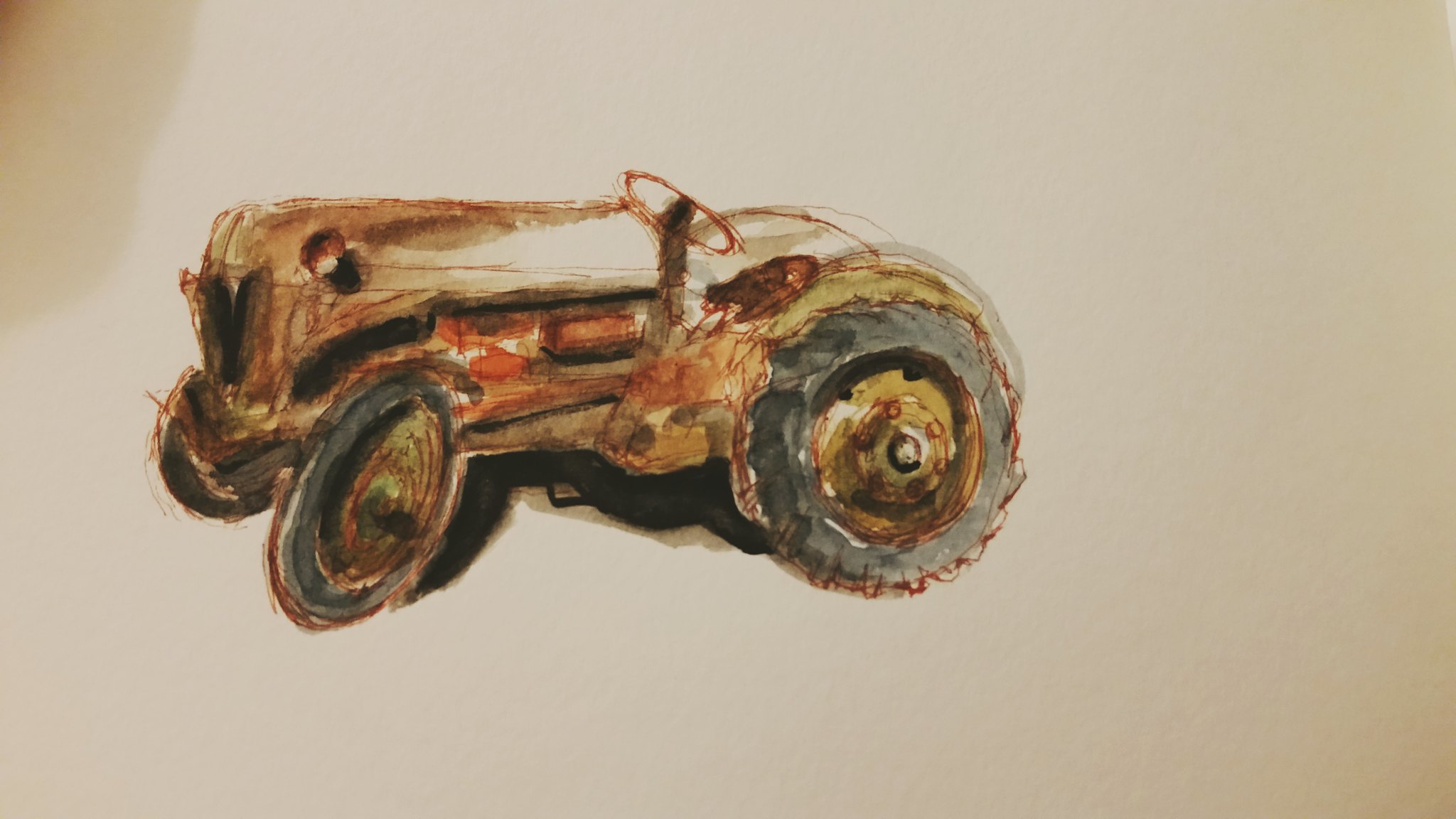This is a detailed watercolor and ink painting of an antique tractor, likely from the 1960s, positioned on a landscape-oriented, off-white sheet of paper with subtle speckles in the background. The tractor, depicted in shades of light brown, dark brown, reds, and rusty oranges, conveys a sense of age and history, with hints of rust suggesting long-term exposure to the elements. The vehicle features a long front end extending to the left, and its tires are painted in grays with greenish-gray rims. The seat is a rusty color, positioned behind the steering wheel, which is also red. There are intricate details, such as lights on the front and a V-shaped design at the end of the hood, likely sketched with a tiny brush or red pen. The scene lacks any additional equipment behind the tractor, emphasizing its solitary, standalone presence.